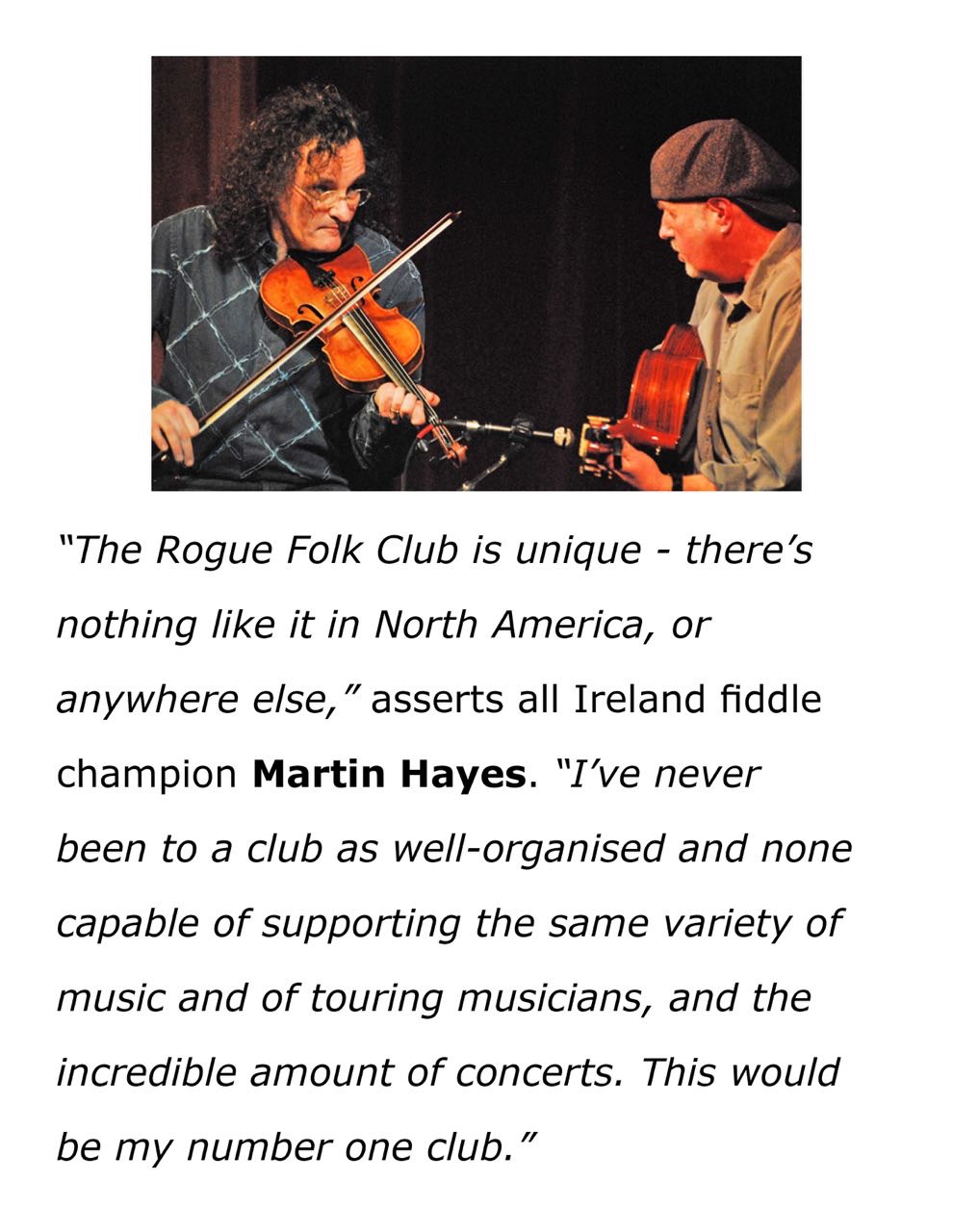The image displays an advertisement or informational piece showcasing The Rogue Folk Club, praised by All-Ireland fiddle champion Martin Hayes. At the top, there's a small picture of two men sitting against a dark curtain. One man, with long, curly brown hair and wearing a blue checkered shirt, is playing a violin. The other man, dressed in a tan button-up shirt with cuffs rolled up and a hat worn backward, is playing an acoustic guitar. The text below the image prominently features a quote in which Martin Hayes, highlighted in bold letters, extols the virtues of the club: "The Rogue Folk Club is unique. There's nothing like it in North America or anywhere else. I've never been to a club as well organized, nor one capable of supporting such a variety of music and touring musicians, and the incredible number of concerts. This would be my number one club."